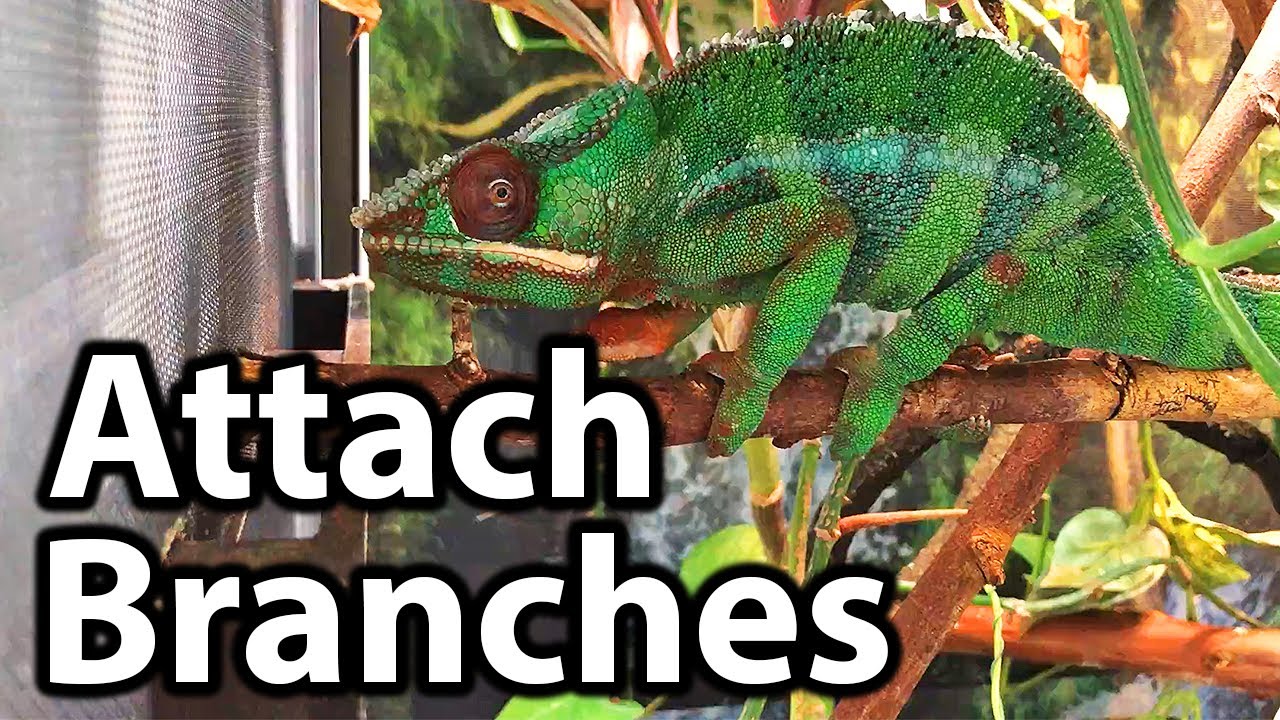The image portrays a widescreen photograph of a lizard, likely an iguana, perched on a branch. The lizard, which some may find unattractive, exhibits a vibrant array of green hues with alternating dark green and light green stripes decorating its belly and body. The photo captures the lizard in a left-profile view, its textured skin and scales clearly visible. Intriguingly, the lizard's left eye seems to be independently rotating towards the camera, adding a curious, almost inquisitive expression to its demeanor. Overlaid on the lower left corner of the image, in large, bold white letters outlined in black, is a text seemingly attached to the branches, split into two lines, providing some sort of descriptive or thematic content. The overall composition spotlights the lizard's unique appearance and captivating presence amidst its natural habitat.